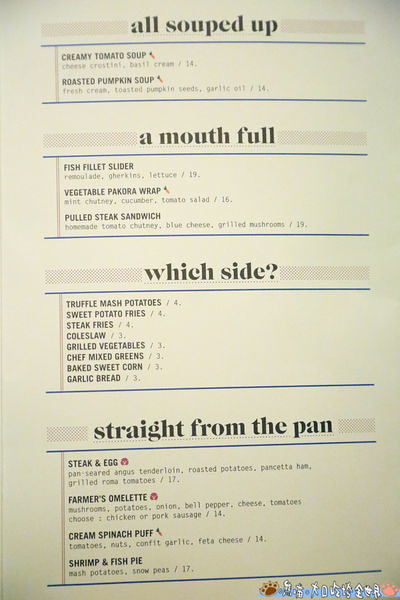The image depicts a clean, minimalistic photograph of a restaurant menu page. The page is white with black text framed by distinctive blue and red borders that form straight lines around each segment of the menu, enhancing its structured layout. Each segment is titled and flanked by small decorative checkered bars.

At the top, the menu is headlined with "All Souped Up" in bold, large letters. This section features offerings such as creamy tomato soup, detailed with cheese crostini and basil cream, priced at $14, and roasted pumpkin soup, served with fresh cream and toasted pumpkin seeds.

Below, the "A Mouthful" section, presumably for appetizers, includes items like fish fillet slider, vegetable pakora wrap, and pulled steak sandwich.

Subsequently, the "Which Side" segment lists a variety of sides, including truffle mashed potatoes, sweet potato fries, steak fries, coleslaw, grilled vegetables, chef’s mixed greens, baked sweet corn, and garlic bread.

Lastly, the "Straight from the Pan" section highlights dishes such as steak and eggs (featuring pan-seared eggs, tenderloin, and roasted potatoes), farmer’s omelet (packed with mushrooms, potatoes, onions, bell pepper, cheese, and tomatoes), creamed spinach puff (with ingredients like tomatoes, nuts, confit garlic, and feta cheese), and shrimp and fish pie accompanied by mashed potatoes and snow peas.

At the bottom of the menu, a small, unexplained paw print is present, adding a curious touch to the otherwise text-focused design.